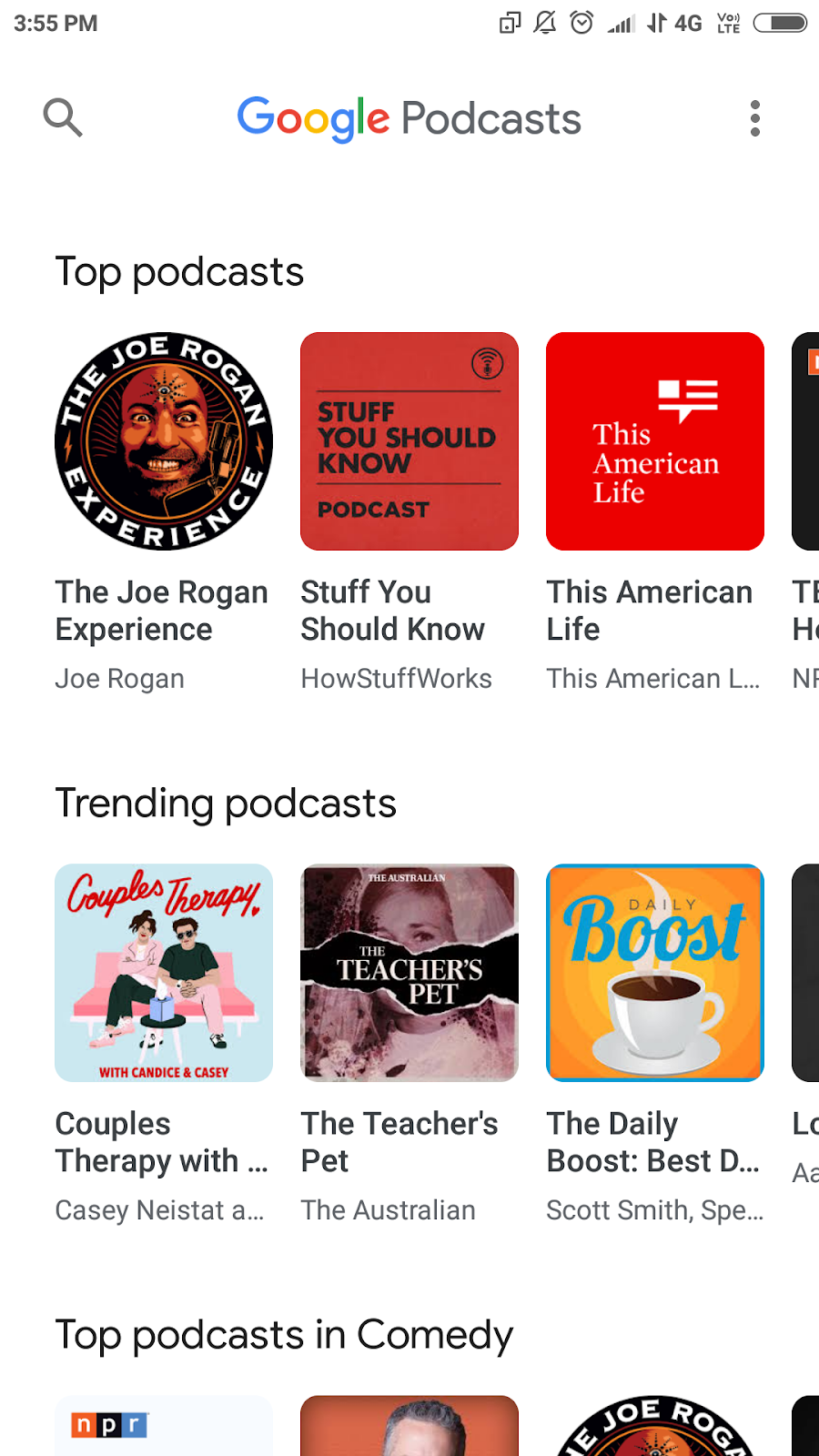The image depicts a cell phone screen showcasing the Google Podcasts app interface. At the top left corner, the time is displayed as 3:55 PM, while on the top right, there are icons indicating no sound, signal strength with 4G LTE, and a battery level at three-quarters full. Below the time, a magnifying glass icon for search is visible on the left. The center of the screen features the text "Google Podcasts," and to the right are three vertically stacked dots signifying a menu.

The main section of the screen is divided into two rows of podcast icons under the heading "Top Podcasts." Each row shows three complete podcast thumbnails with a partially visible fourth one at the far right edge. The podcasts listed in the first row are:
1. "The Joe Rogan Experience" by Joe Rogan,
2. "Stuff You Should Know" by How Stuff Works,
3. "This American Life," abbreviated as "This American L..." due to space constraints.

The second row features "Trending Podcasts" such as:
1. "Couples Therapy" by Casey Neistat,
2. "The Teacher's Pet" by The Australian,
3. "The Daily Boost" by Scott Smith, labeled as "The Daily Boost Best D..." and "Scott Smith, SPE..." due to truncation.

Below these rows, partially visible text indicates a category for "Top Podcasts in Comedy," and faint glimpses of additional icons include "NPR" and a man's forehead. The background is white, providing a clean and straightforward appearance for the app interface.